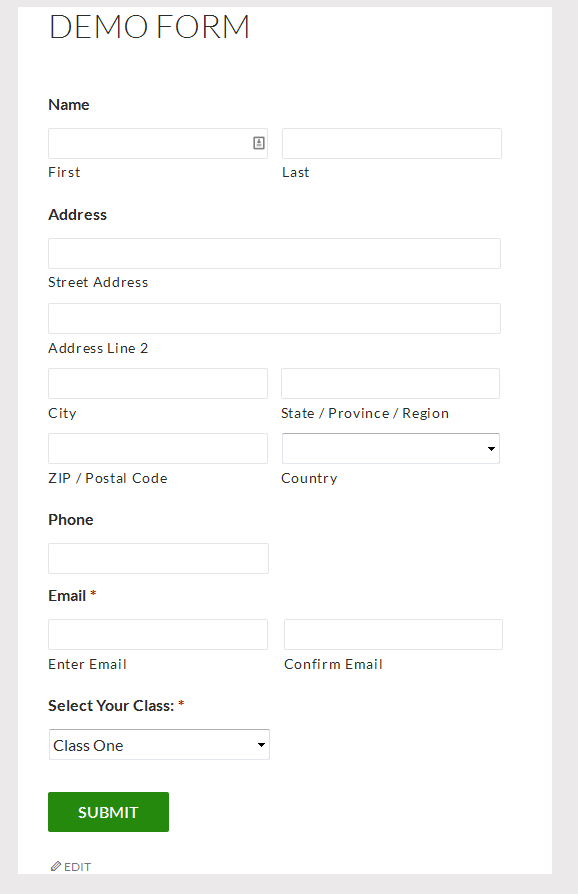The image appears to be a screenshot of an online form titled "DEMO FORM," prominently displayed at the top in capital letters. The form is primarily designed with black text on a white background and is framed by a grey border that is thicker on the bottom and right sides, and thinner on the top and left sides.

The form starts with fields for entering a name, including separate boxes for first and last names, followed by sections for address details such as street address, address line 2, city, state/province/region, and zip/postal code. There's also a dropdown menu labeled "Country."

Next, there are bolded fields for "Phone" and "Email," with a red asterisk next to the "Email" label indicating it's a required field. Users are prompted to enter their email address and then confirm it in a box to the right.

Below the email section, there is another required field marked by a red asterisk: "Select Your Class," accompanied by a dropdown menu with "Class 1" as the default option.

The form concludes with a green "SUBMIT" button on the left side, written in white text. Just above the grey border at the bottom, the word "EDIT" appears in grey, capital letters, accompanied by a small icon of a pen or pencil to its left, indicating an edit option.

Overall, this screenshot likely represents a sample form demonstrating how to design a customizable form using specific software.